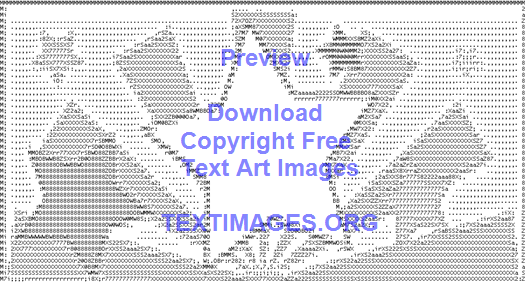The image displays a piece of ASCII art set against a white background with light gray shading. The central focus is a large, pixelated star composed of variously shaded characters, numbers, and symbols, giving it a detailed and nuanced appearance despite lacking straight lines. Surrounding this main star are several smaller stars with varying degrees of opacity, creating a dynamic burst effect. Blue text overlays the image, reading: "Preview Download Copyright-Free Text Art Images textimages.org." The shading and detail are achieved solely through the clever arrangement of keyboard characters, contributing to its intricate and realistic look.